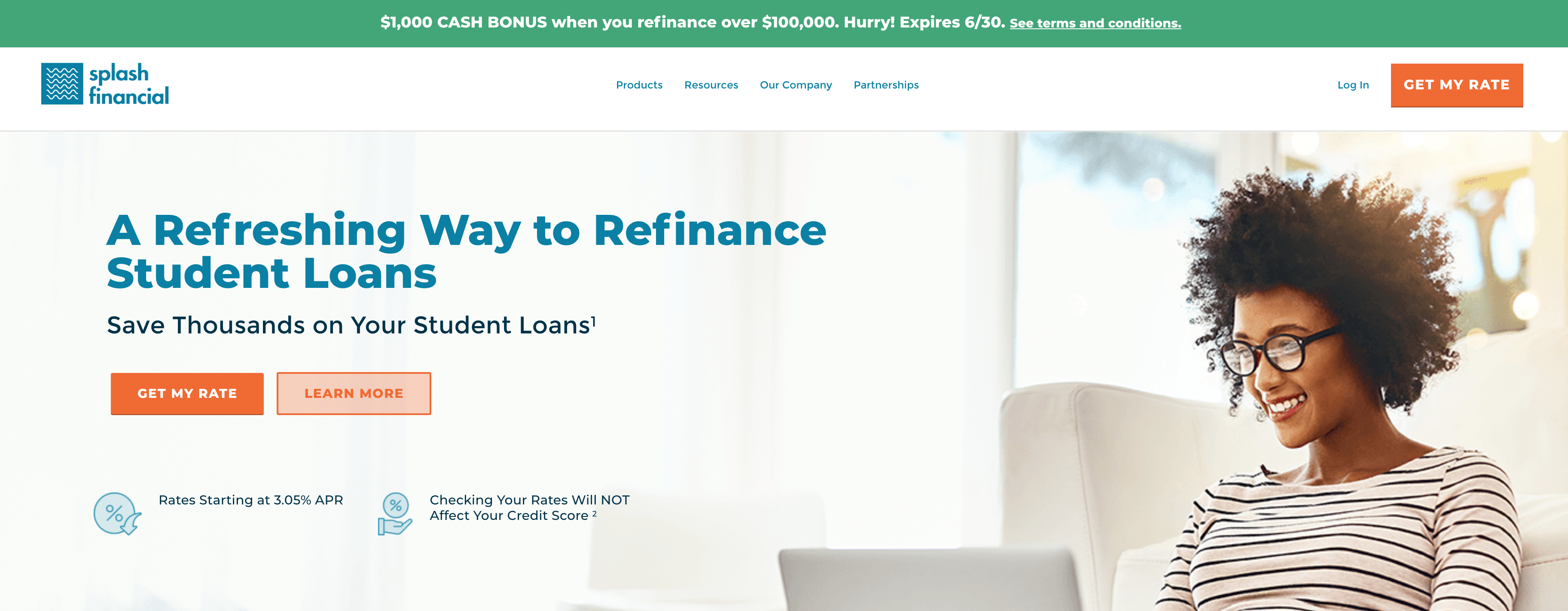The screenshot features a detailed promotional banner for a refinancing service, presented in a horizontal rectangular shape. At the top, a green banner spans the width of the image, prominently displaying the text "$1000 Cash Bonus" in white, with "Cash Bonus" capitalized. This promotional offer states "When you refinance over $100,000" and adds an urgency with the message "Hurry! Expires 6-30." Below this, a sentence in very small, unreadable text is present.

The main body of the image is divided into two sections. On the left, the background is white. A blue square is positioned near the top left corner, to the right of which the word "Splash" appears, followed by "Financial" in bold blue font beneath it. Four blue words are centered directly below this text.

On the right, occupying about half of the screenshot, a red rectangular button labeled "Get My Rate" in white text captures attention. Below this button, a larger section features a photograph of a smiling Black woman with spiky dark hair and wearing dark glasses. She is seated on the floor, leaning against a white couch, and is focused on a gray laptop. The woman is dressed in a white long-sleeved top with horizontal black stripes.

To the left of the woman's image, two text blocks are present. The top block in blue states, "A Refreshing Way to Refinance Student Loans," followed by a black text block that reads, "Save Thousands on Your Student Loans." Below these text blocks, two rectangular buttons are aligned in a row. The left button is orange and says "Get My Rate" in white text, while the right button is a lighter shade of orange with the text "Learn More" in bold orange.